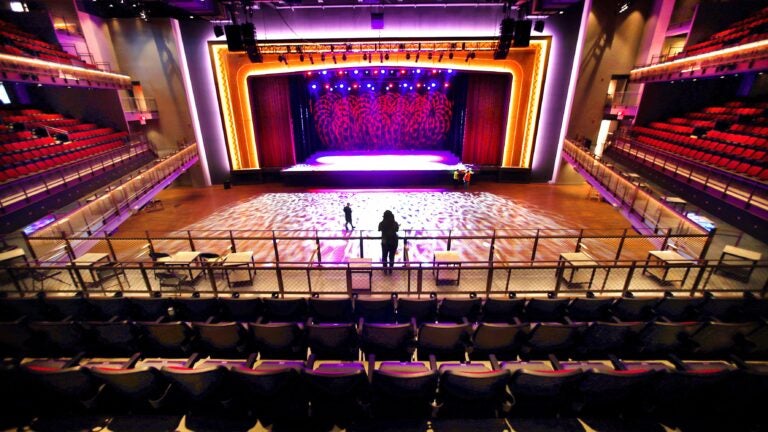The image captures an empty stage in a theater-like setting, adorned with an array of blue, red, and white lights creating a vivid atmosphere. The stage features a striking red curtain as its border, against a reddish-black backdrop, with additional lights mounted at the top. In front of the stage, there's a well-lit wooden area, potentially a standing room section, encircled by railings. The auditorium is filled with rows and rows of red cushioned seats that can be folded up.

On the stage, there are three people: two positioned near the front and one towards the back, all seemingly engrossed in observing their surroundings. Additionally, a person stands by the red seats and a pathway that loops around in a square shape, giving structure to the seating arrangement. Another individual is seen on the balcony, also looking towards the stage. The scene conveys a sense of calm and introspection, as if the people are taking in the ambiance without the pressure of an active performance or an audience. The overall mood suggests a moment of quiet preparation or admiration of the theater setting.